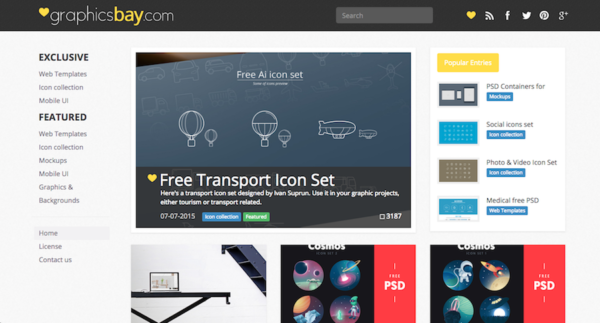This caption has been rephrased and structured for clarity and detail:

---

The top section of the page for GraphicsBay.com features a striking black bar. On the left side, there's a small yellow heart icon followed by the site’s name, GraphicsBay.com, with the word "Bay" highlighted in yellow. Progressing to the right, there is a search bar accompanied by various icons, including a yellow heart, Facebook, Twitter, Pinterest, and Google Plus.

Below this section, the background transitions to light gray. On the left side, written vertically, are the words "Exclusive" in bold type, followed by "Web Templates," "Icon Collections," and "Mobile UI," all in gray.

Directly to the right, the title "Featured" is prominently displayed in bold black letters. Beneath this, a list in gray text includes "Web Templates," "Icon Collection," "Mock-ups," "Mobile UI," "Graphics," and "Backgrounds," arranged from top to bottom.

Further down, navigation links for "Home," "License," and "Contact Us" are positioned. At the very bottom center of the page, a vibrant blue box labeled "Free AI Icon Set" is displayed, accompanied by unreadable text. Beneath it, icons reminiscent of hot air balloons and a zeppelin are visible. Following this, a section titled "Free Transport Icon Set" includes additional unreadable text, a date, and blue and green boxes.

Below these elements, there is a white section, possibly part of stairs with a laptop placed on a table. Adjacent to this, another icon section labeled "Cosmos" showcases colorful planets. Next to this, in a red box, the initials "PSD" are noted. 

On the far right, a yellow box at the top contains unreadable text, followed by four distinct sections labeled "PSD Containers for Social Icons," "Photo and Video Icon Set," "Medical Free PSD," and another icon section similar to "Cosmos with Planets" but including a red part that also reads "PSD."

---

This detailed description encapsulates the various elements and layout of the page, providing a clear and comprehensive view.